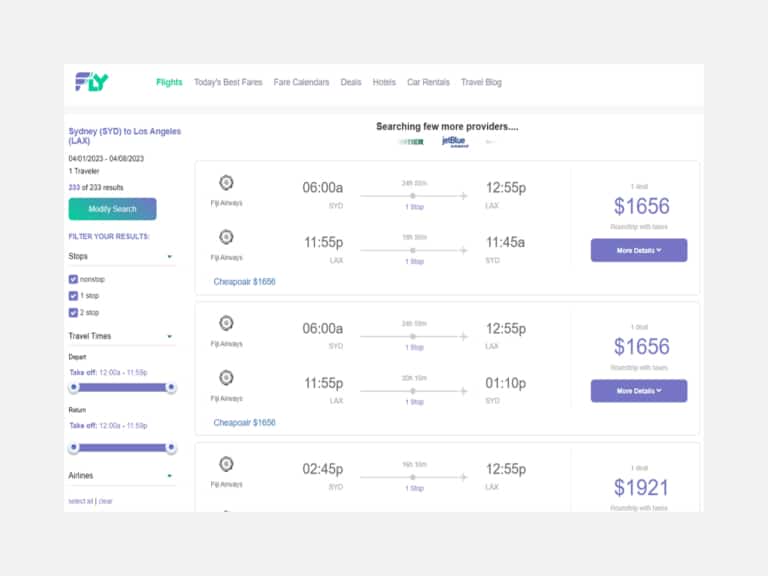A square screenshot features a user interface with a grey background, upon which is superimposed a white square. The top left corner prominently displays the Fly logo, followed by the word "Flights" in green text to its right. Adjacent to this are navigation options: "Today's Best Fares," "Fare Calendars," "Deals," "Hotels," "Car Rentals," and "Travel Blog." 

On the upper-left section of the screenshot, there is detailed trip information indicating a flight from Sydney to Los Angeles. This is accompanied by travel dates, the number of travelers, and a summary of available search results. Below this, a "Modify Search" button allows users to adjust their search criteria, followed by an option to "Filter Your Results."

To the right, flights are listed diagonally down the page, each entry providing departing and arrival times for round trips. Corresponding prices are displayed to the right of these times, with an accompanying "More" option in a purple bar for additional details. To the left of each flight listing is the airline's logo, with a note indicating "Cheaper, Cheap Air price" below it.